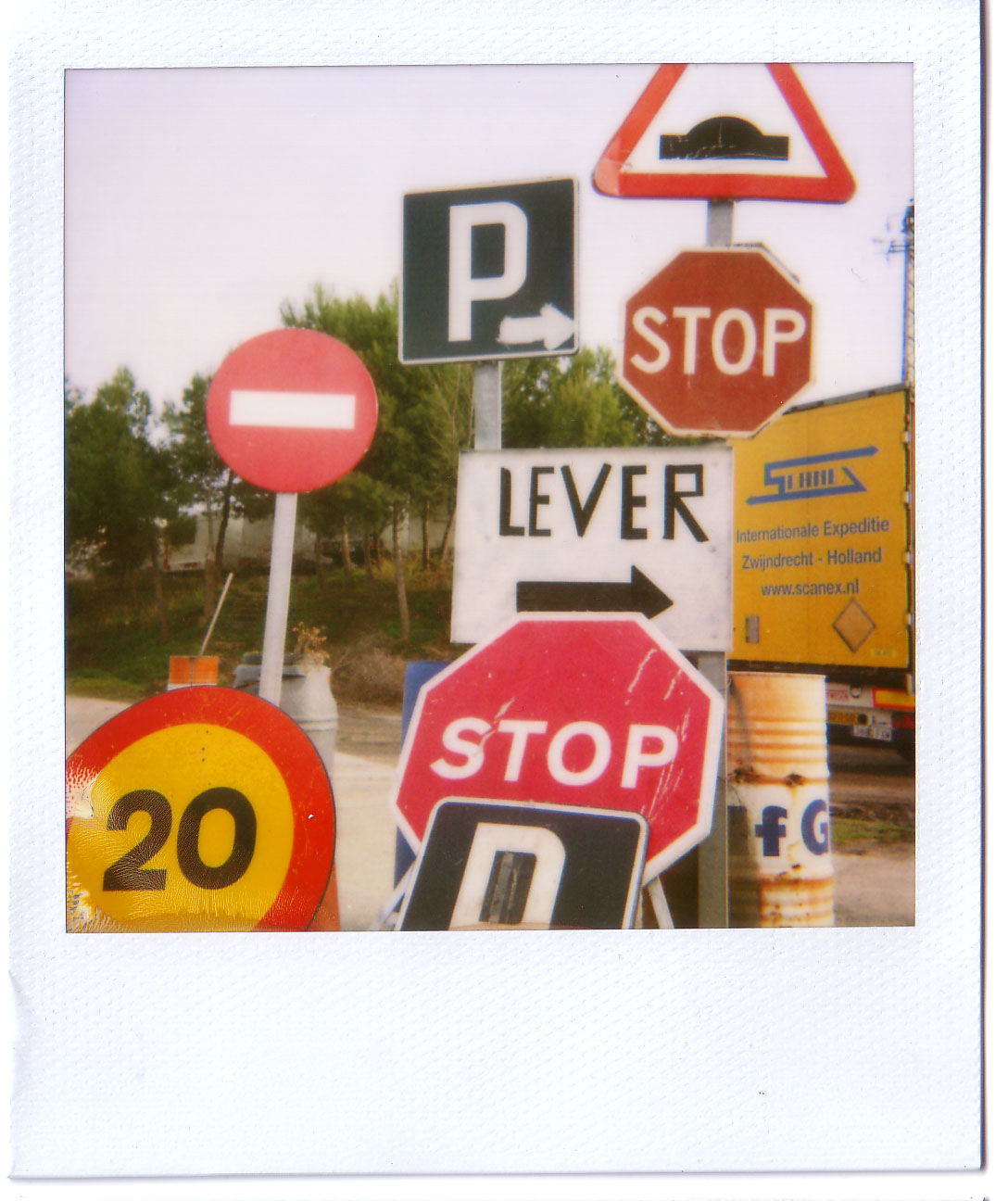This Polaroid photograph, slightly bent on the left side with a rough-textured white frame, captures a clutter of diverse street signs set against an outdoor, daytime backdrop with green trees and a gray-tinted sky. At the top, a triangular sign with a red border and a partially visible black symbol (possibly a stylized car) is prominently featured. Below it hangs a classic red stop sign with white text. Adjacent to these is a white sign reading "LEVER" in black letters, accompanied by a right-pointing arrow. Further down, a black sign with a white 'P' and an arrow points to the right. To the left, a circular red sign bears a white horizontal stripe, resembling a 'no entry' sign, while beneath it, another round sign has an inner yellow circle with the black number '20' at its center. Another yellow rectangular sign with blue text reads "Internationale Expeditie Zwijndrecht Holland" followed by "www.scanx.nl," indicating a Dutch origin. Scattered among these signs, a rusty, pinkish-orange oil drum marked with blue letters "F" and "G" and a metal barrel with indistinct markings can be seen. All signs are tightly packed, creating a chaotic yet intriguing scene. A building is faintly visible behind the trees at the back, suggesting the setting might be in a park-like area.